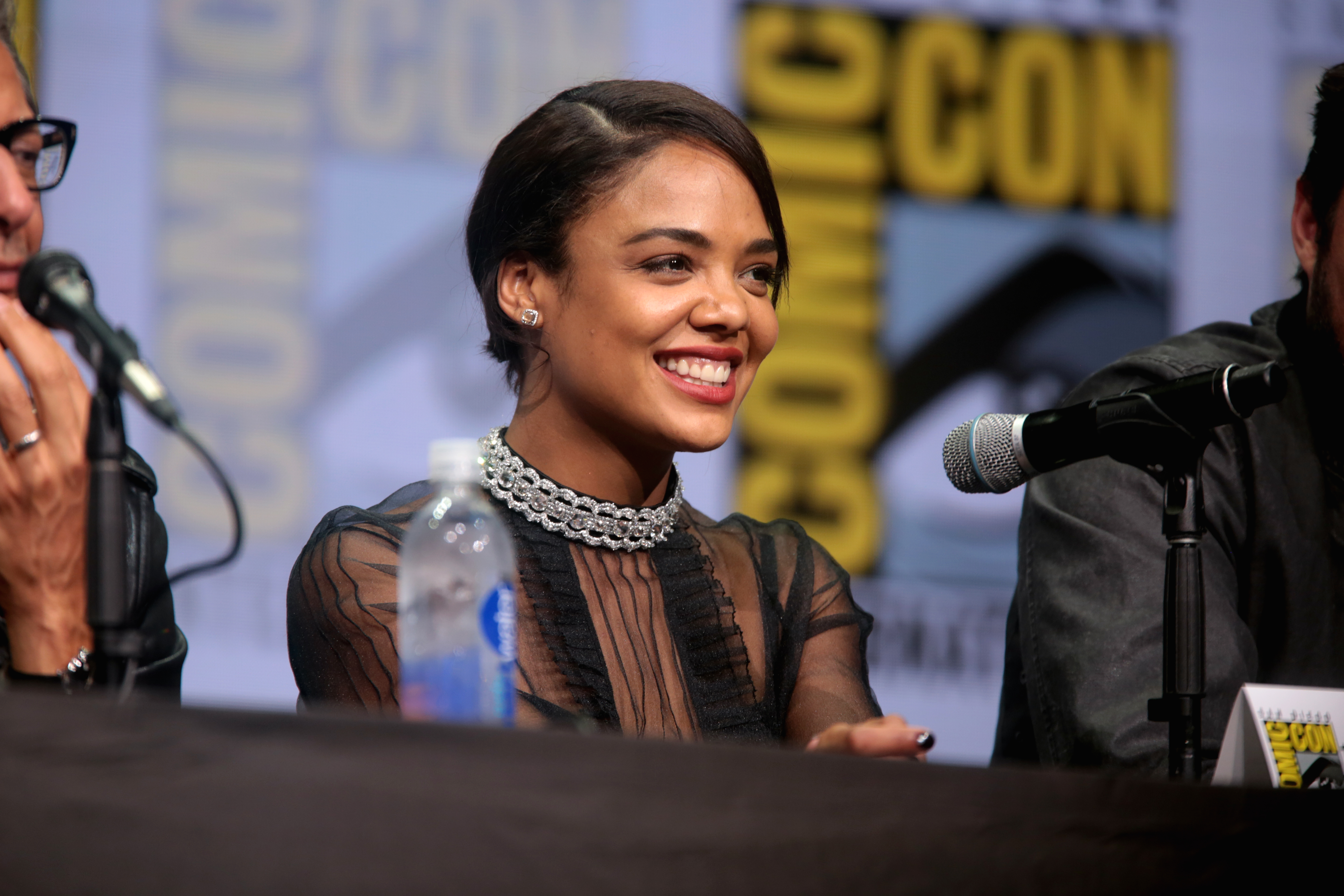In the center of this indoor image, taken at a Comic-Con event, actress Tessa Thompson is seen smiling while seated at a black table, participating in a panel discussion. She is positioned directly in the center, flanked by two male individuals. Tessa is wearing a sheer black shirt with thick black stripes on the front and a thick, gym-studded silver choker necklace. In front of her on the table is a microphone and a bottle of vitamin water. The backdrop features a blurry Comic-Con banner, recognizable by its distinct upside-down L shape, yellow and black color scheme, and illustrated eye with a dark eyebrow above it in a blue color scheme. The scene includes a variety of colors including black, white, gray, silver, light blue, yellow, blue, and brown. A tablecloth-covered table is visible at the bottom of the frame, completing the setup typical of a convention setting.